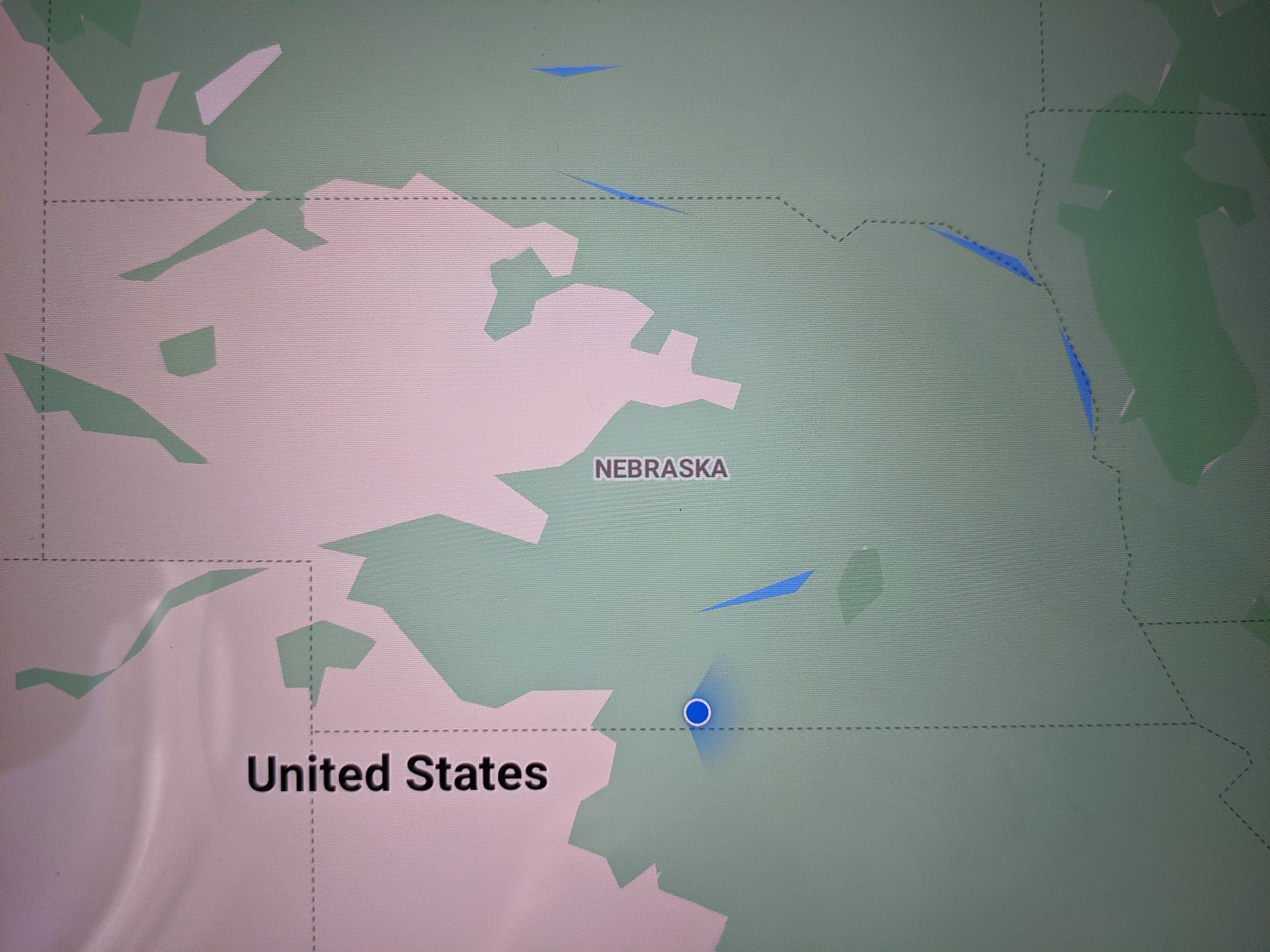The image is a graphical illustration of a map featuring a portion of the United States, prominently highlighting Nebraska. The base of the map is predominantly light green, overlaid with sections of pink, although the significance of these colors is not elucidated. Nebraska stands out as the only labeled state, its name presented in bold, black capital letters with a distinct white outline. The map includes dotted lines to signify state boundaries, with a notably thicker dotted line demarcating Nebraska’s southern border. Towards this southern edge, there is a distinctive blue dot encircled by a white ring, emanating a radar-like symbol indicative of a navigation app marker. Sporadically scattered across the map are irregular blue streaks, which are narrow and triangular, defying typical depictions of water bodies. Additionally, a patch of darker green appears towards the top right corner of the map. The overall layout includes the text "United States" in a prominent font size situated in the bottom left corner, contrasting sharply with the Nebraska label.